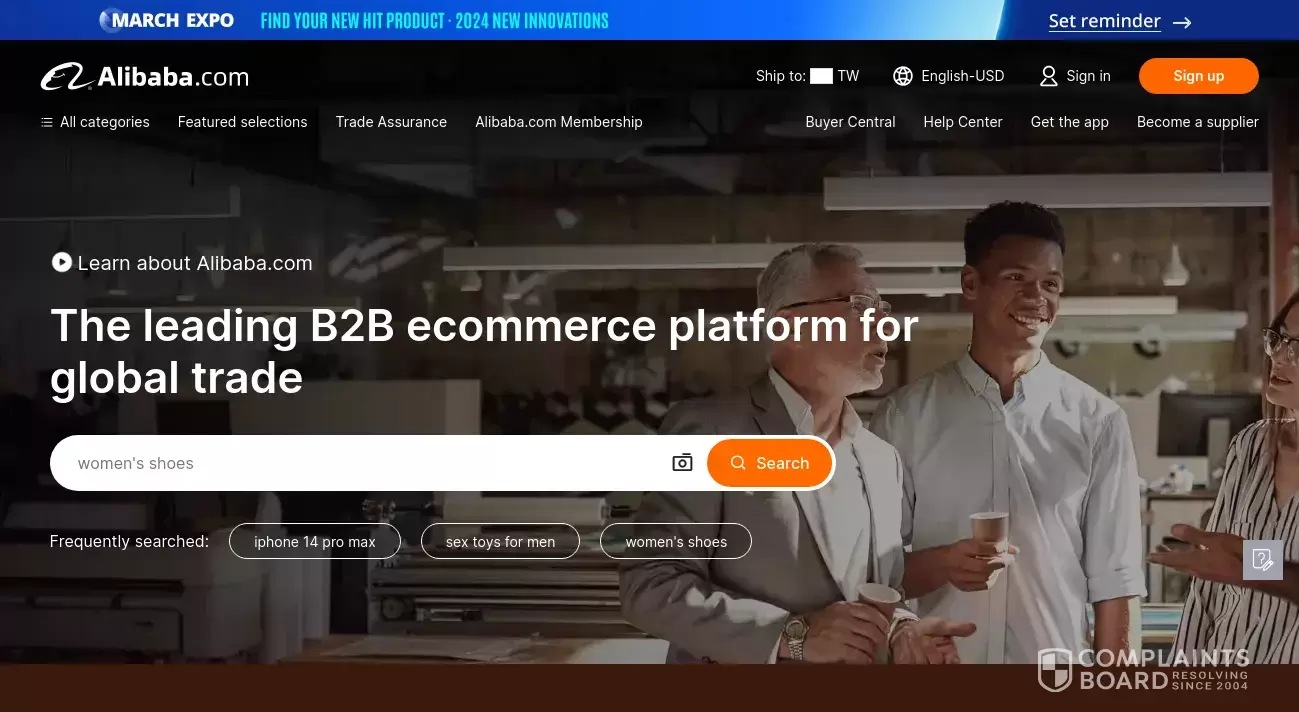The image displays a detailed screenshot from a webpage, prominently featuring a blue banner across the top. In bold white text, the banner announces "March Expo," followed by the tagline "Find your new hit product" and "24 new innovations." Toward the upper right corner, positioned against the dark blue section, there is a "Set Reminder" button accompanied by a right-pointing arrow for added visibility.

Below the banner on the top left, against a black background, the Alibaba logo is prominently displayed alongside the text "Alibaba.com." Just beneath this, a slogan in large bold white text reads, "The leading B2B e-commerce platform for global trade," highlighting the platform's prominence in international business. 

Further down the image, there is a functional search bar, pre-filled with the search term "women's shoes." Accompanying the search term is a small camera icon positioned within the search bar and a search button ready for interaction. The overall layout and text are designed to guide users through discovering new products and engaging with Alibaba’s expansive B2B marketplace.